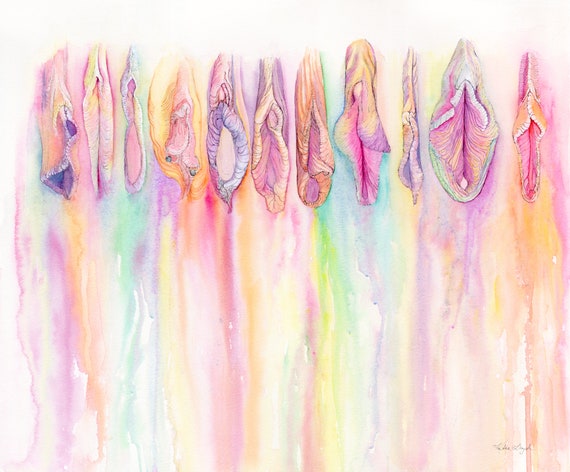This watercolor painting displays 11 distinctive depictions of female genitalia, each presenting a unique style and anatomy from left to right across the top of the canvas. Rendered in an array of pastel hues—including pinks, greens, yellows, oranges, and purples—these varied illustrations highlight differences such as open or closed labia, wrinkled vs. flat textures, wide vs. small shapes, and coverage of the clitoris. The delicate watercolors drip downward, creating a flowing, rainbow-like effect as the colors blend together. In the bottom right corner, the artist has signed their name in pencil, completing the composition.